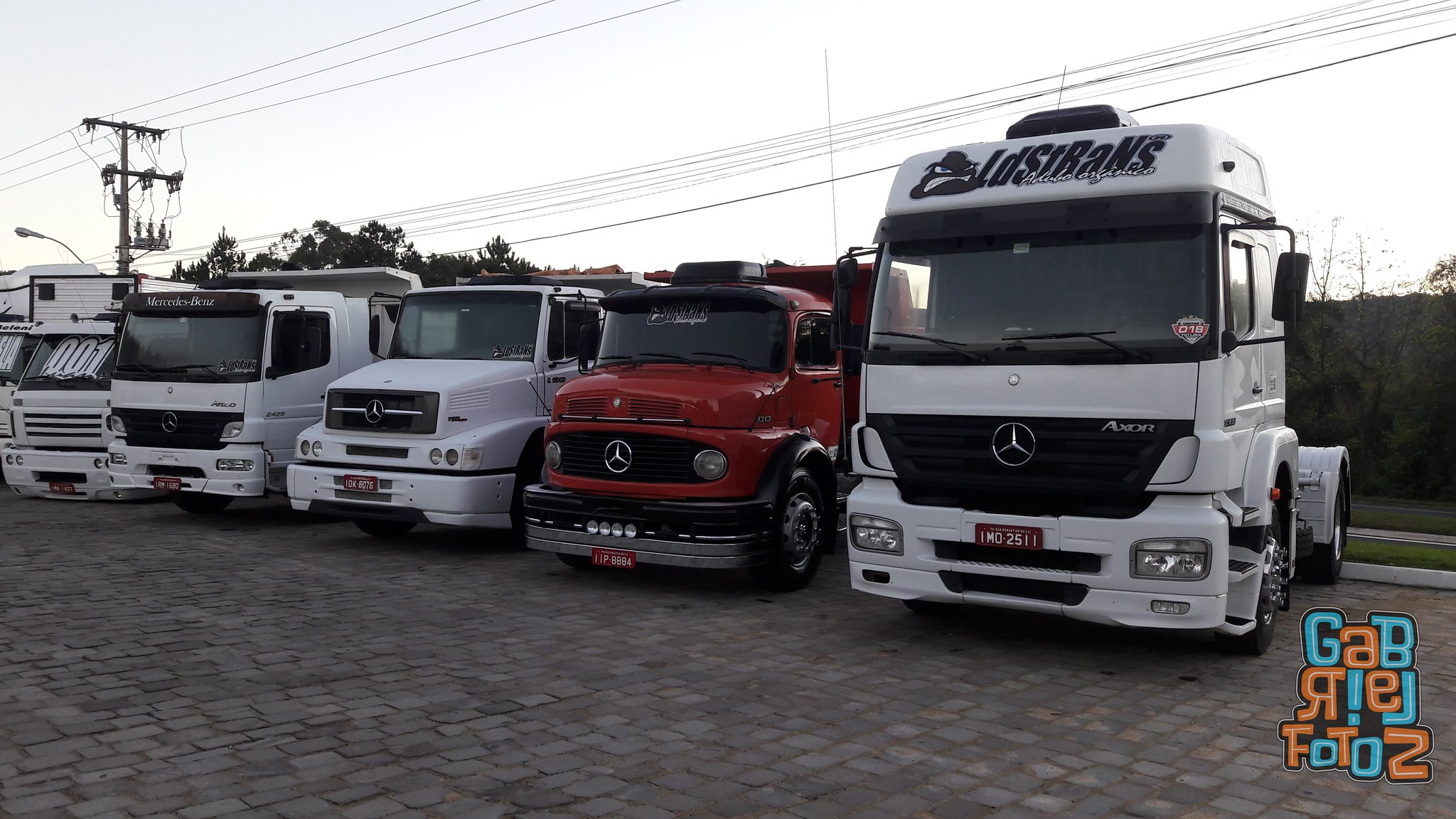The outdoor image depicts a lineup of five larger vehicles parked in a bricked parking lot, facing the camera. The vehicles appear to be mostly Mercedes-Benz trucks, as evidenced by the iconic Mercedes emblem on their front grilles. Starting from the right, the first vehicle is a white Mercedes-Benz semi-truck cab with a black grille. This truck does not have its bed attached, displaying only the front part where it would typically connect. There is a sticker on the windshield and an inscription on the pop-up area, reading "ID Strands" and depicting an angry bulldog.

Next to it, on the left, is an older red vintage Mercedes truck, possibly a dump truck with a small cabin and a noticeable brown license plate. Following this is another white Mercedes truck, slightly newer with an extended hood, maintaining the signature emblem on the front. Adjacent to it is a boxier white Mercedes truck with a flat, square face. This vehicle, too, bears the Mercedes logo and has “Mercedes Benz” lettering on the top of the windshield.

The fifth vehicle on the far left stands out as it appears to be an RV and does not feature the Mercedes emblem. Instead, it is grounded with no visible wheels and has "001" displayed in its window in white numbers.

Behind this row of vehicles, a green fence or wall made of plants and bushes is visible, along with some dry trees or plants and a utility pole with power lines crisscrossing the sky. The photograph is clearly taken during the daytime under the brightness of natural sunlight. In the bottom right corner of the image, the watermark "Gab Real FOTOS" in blue and orange letters, adds a notable detail to the scene.